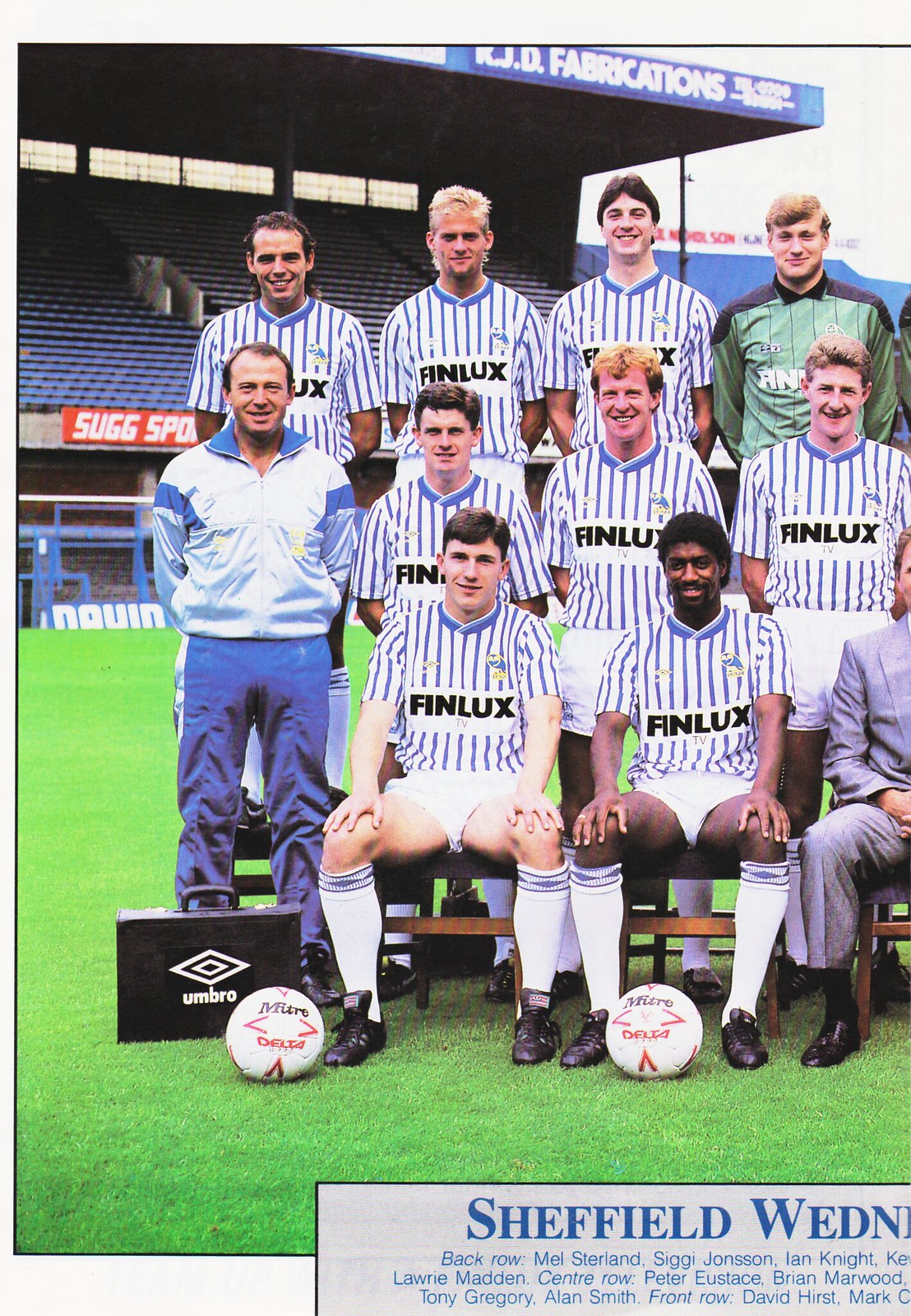In this vibrant photo, a group of Sheffield-based male soccer players and their coach pose outdoors on a lush green field, likely artificial turf. They form three discernible rows: the front row is seated on a wooden bench, the middle row stands directly behind them, and the back row stands elevated on another bench. All the players don a consistent kit featuring white jerseys with blue stripes, white shorts, high white socks, and black boots. Notably, the goalkeeper wears a distinguishing green jersey with black shoulders. The team’s trainer stands out in a white and blue windbreaker paired with blue pants.

In the back row, from left to right, the first player in the white and blue striped jersey has dark hair, followed by a blonde-haired player in the same outfit. Next to him is a player with centrally parted black hair, and then a player with light brown hair in the green goalkeeper's jersey. The middle row includes an older man in the white windbreaker with blue accents, standing among players with varying shades of brown and dark hair, all in the team jersey. 

The front row, seated, features a man with black hair parted on the right, wearing the same team jersey with "FINLUX" emblazoned across the chest. Beside him, a black player also in the team uniform, both with hands on their knees. Partially visible, the next person is clad in a gray suit with clasped hands on his lap. A distinct text at the bottom reads "Sheffield W-E-D-N," which is cut off, suggesting it names the team or club. Below the group, labeled rows reveal player names: Black Row includes Mel Sherlyn, Siggy Johnson, Ian Knight, Lane Madden; Center Row includes Peter Eustace, Brian Marwood, Tony Gregory, Alan Smith; Front Row features David Hurst and Mark. The background showcases stadium bleachers with blue seats and a banner reading "KJD Fabrications." Another banner below the first level displays "S-U-G-G-S-P-O." The ground in front hosts two white soccer balls with orange and brown lettering. A black suitcase bearing a diamond logo labeled "UMBRO" rests at the bottom left.